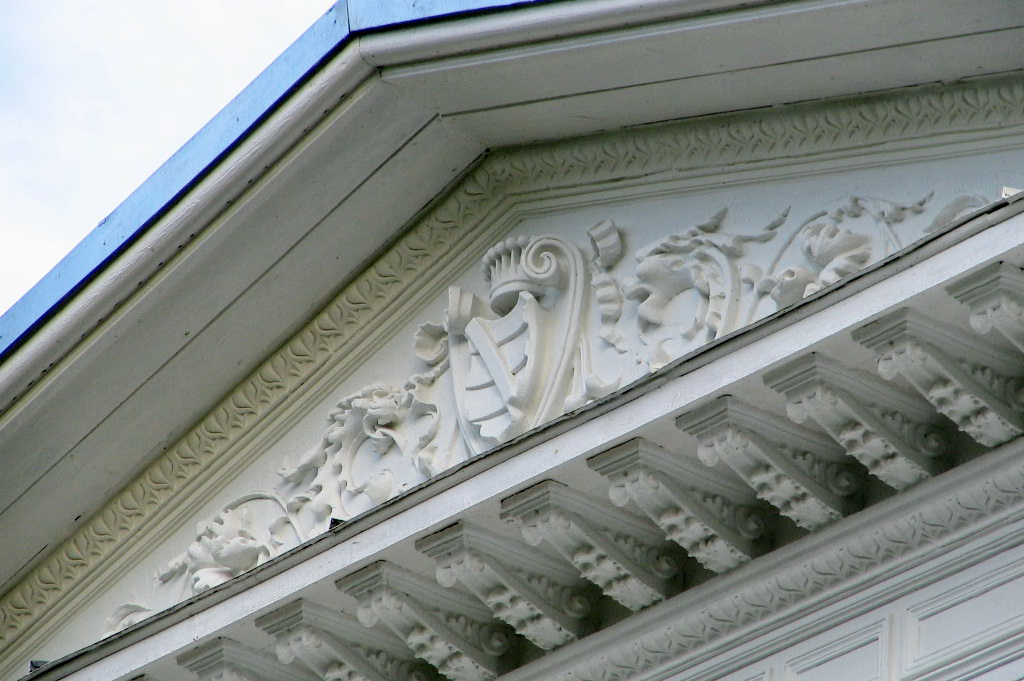The image depicts a close-up of the ornate eave of a building's rooftop, showcasing intricate architectural details. The rooftop itself is a bluish metal, atop a layer of gray wood or similar material. The structure features Victorian-style crown molding with scrolling leaves and dragon heads, executed in a white, stucco-like material. At the apex where the A-frame meets, a carved crest with a crown and shield is centered, with dragons facing towards the crown, which has multiple points capped with circular embellishments. Below the crest, a black metal band traverses the eave, supported by elaborate beams and rectangular multi-level carvings, all maintaining a cohesive white color scheme. The backdrop reveals a triangular slice of the cloudy sky, adding a contrasting element to the detailed decor of the building’s topmost section.